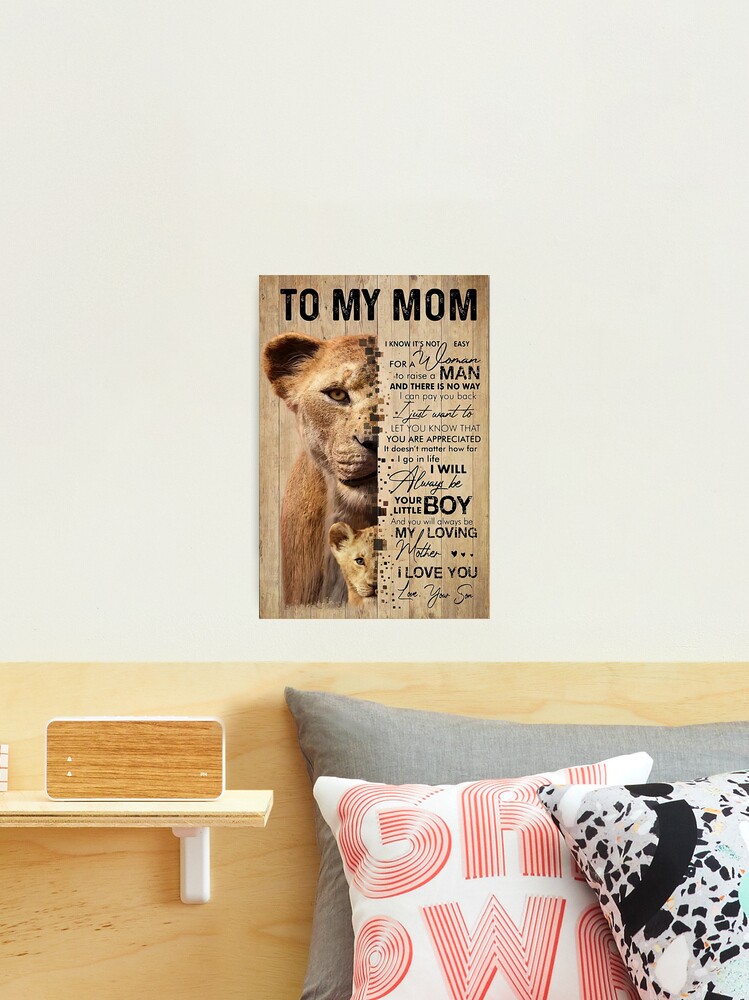The close-up image shows a section of a bedroom wall, primarily focusing on the headboard and a framed poster in the center of the wall. The wall is a light green-gray color. The prominently placed poster measures approximately 8x12 inches and features the heartfelt message "To My Mom" at the top. The left side of the poster showcases the profiles of an adult lion and its cub, both cut in half and staring forward. The right side is adorned with various loving messages from a little boy to his mother in different scripts, including phrases like “I will” and “I love you.”

Beneath the poster is a headboard made of light oak wood, which has a pressed wood shelf attached to it. On the shelf lies an oak Bluetooth speaker that adds a rustic touch to the setup. The bed is adorned with three pillows: a gray pillow placed at the top, a white pillow with the red letters "GRL PWR" (omitting the vowels), and a white pillow with a black webbing pattern. The overall ambiance of the image conveys a mixture of heartfelt sentiment and cozy decor.